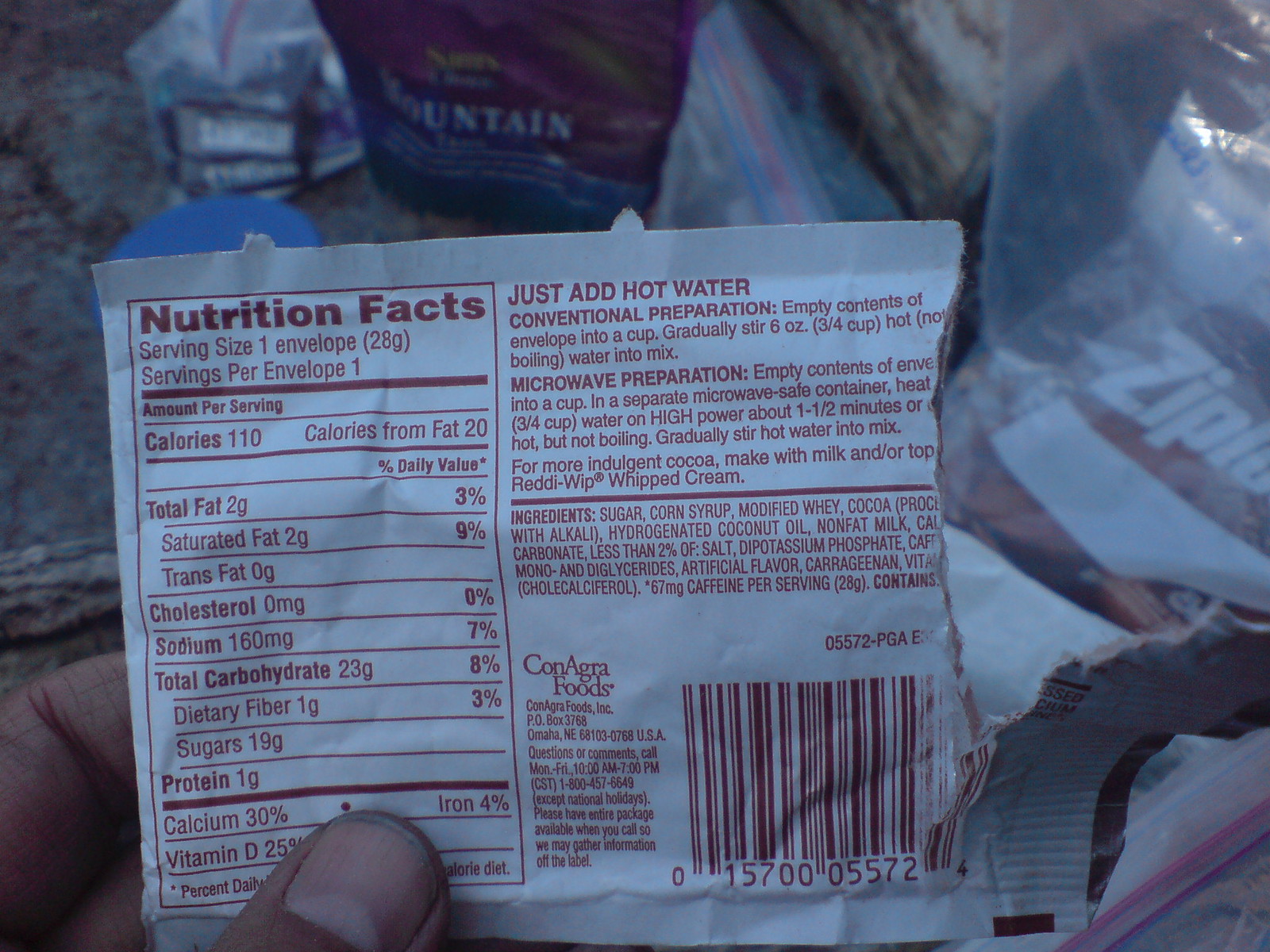In this image, a white paper package of a food product is held in someone's left hand, positioned prominently in front of a countertop cluttered with various other packages and plastic bags brimming with food items. The package, which appears to be slightly larger than a bank card, is visibly torn open on its right side. The exposed top reveals that it has been previously opened, likely to pour out its contents. The label on the package showcases nutrition facts, preparation instructions, ingredients, copyright details, and a barcode. Given the first few ingredients listed—sugar, corn syrup, modified whey, and cocoa—it is plausible that the package contained a sugary substance, possibly a type of sweetener or a dessert mix.